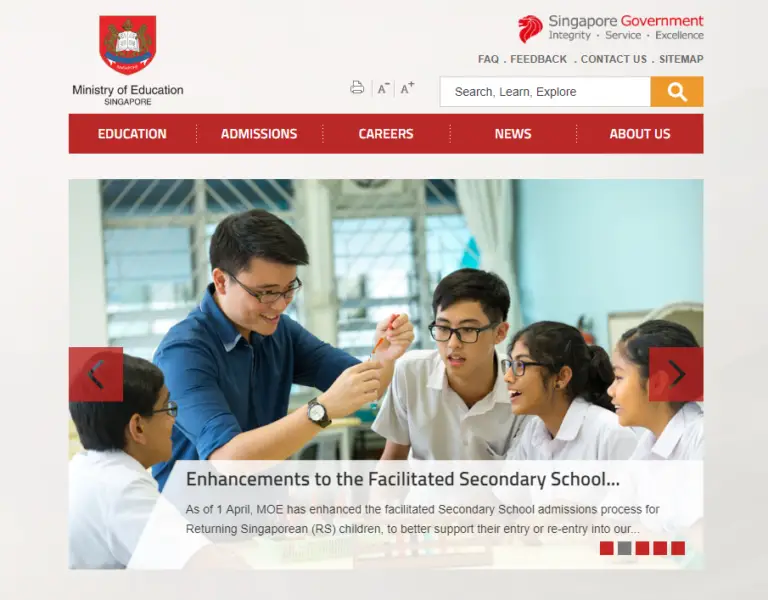A small screenshot of a website belonging to the Ministry of Education in Singapore. In the upper left corner, the Ministry of Education’s name is written in black text. Directly above this, the school's icon is prominently displayed; it features a shield-shaped emblem with a red background. Flanking the emblem, there are two gold lion figures, each holding an open white book. Below them, a blue, upturned, and curved banner can be seen. 

The website's background is light gray. On the right side, information about the Singapore government is displayed, with "Government" written in red. Underneath, the values "Integrity, Service, Excellence" are listed. Beneath these values, there are several clickable links - FAQ, Feedback, Contact Us, and Sitemap. Below these links is a white, rectangular search bar accompanied by an orange, rectangular search button adorned with a white magnifying glass icon.

Further down, the website features a long, rectangular menu with a red background and white text, listing categories such as Education, Admissions, Careers, News, and About Us. Below this menu, there is an image depicting a classroom setting. A teacher dressed in a blue shirt, with short black hair and black glasses, is shown injecting a substance into a test tube while four students observe attentively.